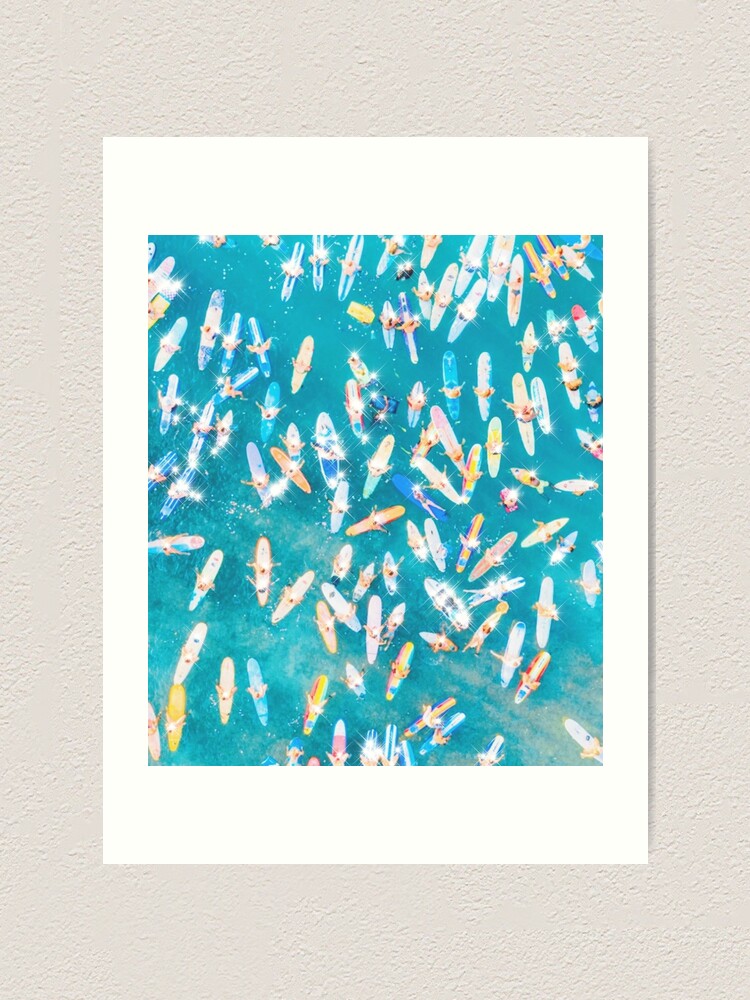The image depicts a vibrant painting of numerous paddle boards scattered across a strikingly clear blue ocean, viewed from above. This detailed artwork captures around 50-60 individuals standing on their boards, each adorned in varied, colorful attire. The paddle boards themselves are painted in vivid colors like white, blue, yellow, and tan, adding to the scene's dynamic composition. The water, almost transparent with glistening white streaks, enhances the painting's tranquil and captivating appearance. The painting, seemingly printed on white poster paper, is framed by its eggshell-colored or taupe backdrop, giving the entire piece a cream-like aura. The scene remains stationary, with the paddle boards mostly aligned in the same direction, and a few oriented differently, depicting a serene, leisurely moment on the ocean.